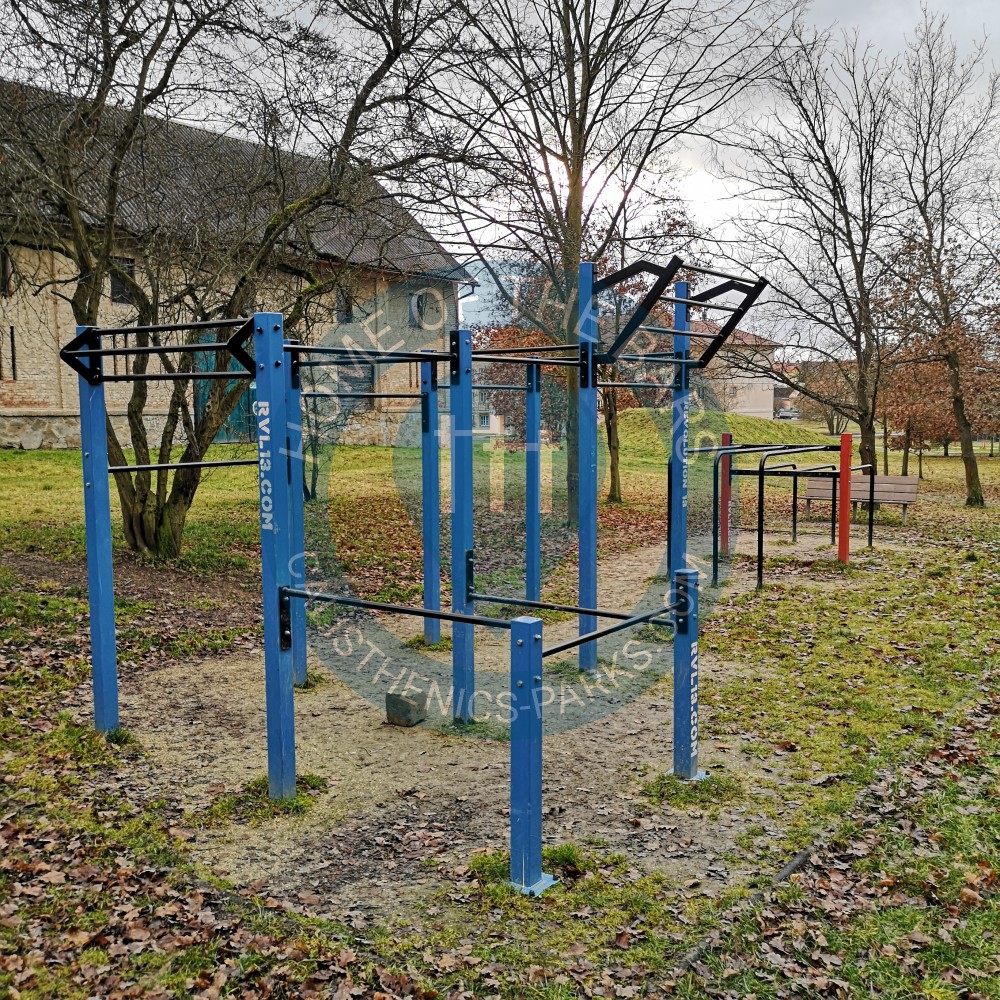This photograph captures an outdoor exercise area that resembles a blend between a playground and a gym, designed primarily for adults. On the left side, blue poles form a structure equipped for exercises such as pull-ups, interconnected by black bars. To the right, a pair of red poles possibly marks an entrance, with black poles situated between them. The blue poles feature the partially visible text "rvl13.com." A watermark reading "Home of the Bars" and "calisthenicsparks.com" is also present, though somewhat indistinct. The surrounding environment indicates a park setting with partially dead grass and spindly, leafless trees, suggesting a fall or winter season. In the background, a building with a dark grey, hipped roof and tan walls stands, under an overcast sky.